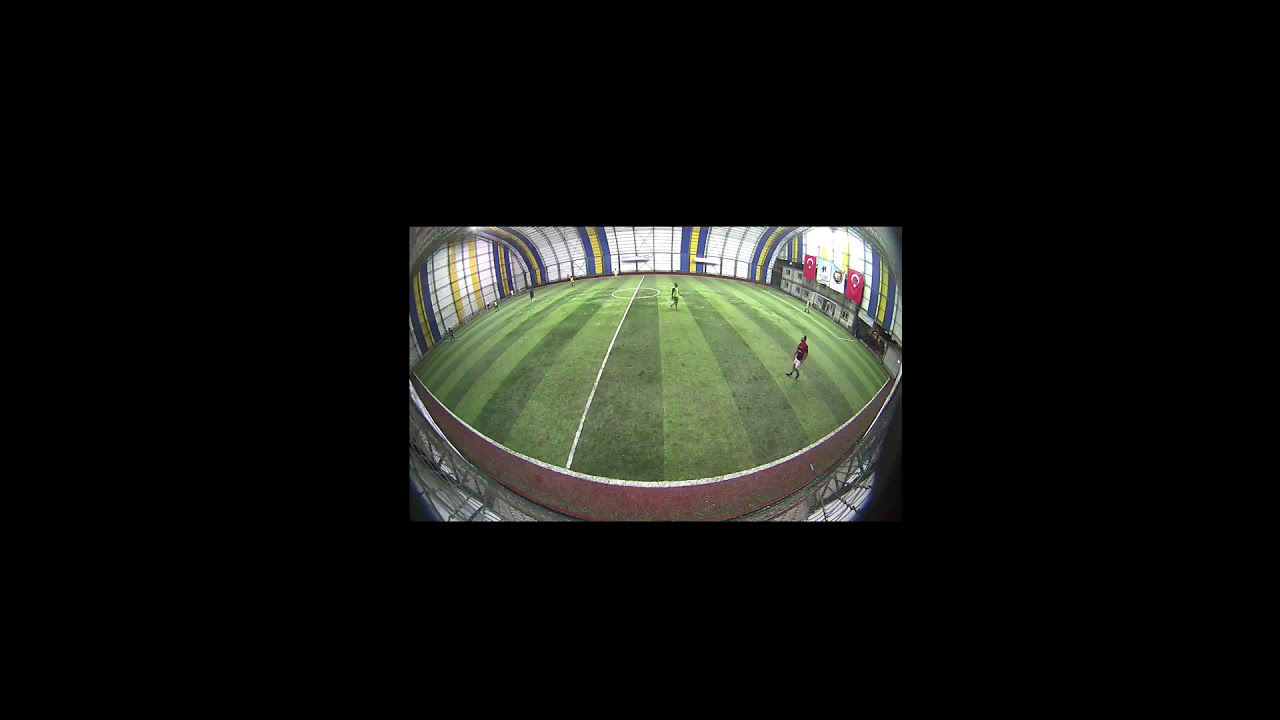The photograph captures an indoor sporting arena with a meticulously maintained green field, featuring alternating dark and light green stripes. The arena is enclosed within a glass-pane dome, giving it a distinct, sometimes eye-shaped appearance due to the wide-angle lens used for the photo. The walls surrounding the field are adorned in white, goldish-yellow, and royal blue hues. A gentleman in white shorts and a reddish top stands prominently in the foreground, while there are additional players and red-and-white items hanging on a wall behind him. A white line runs down the center of the field. The structure's dome, composed of square glass panes, curves around the perimeter, creating a panoramic enclosure. In the upper right-hand corner sits what appears to be a scoreboard. The surrounding metal structure can be glimpsed on both the bottom left and right sides of the frame. The overall image, framed in black, appears small on a 1080p screen, enhancing the compact and detailed view of the indoor arena.